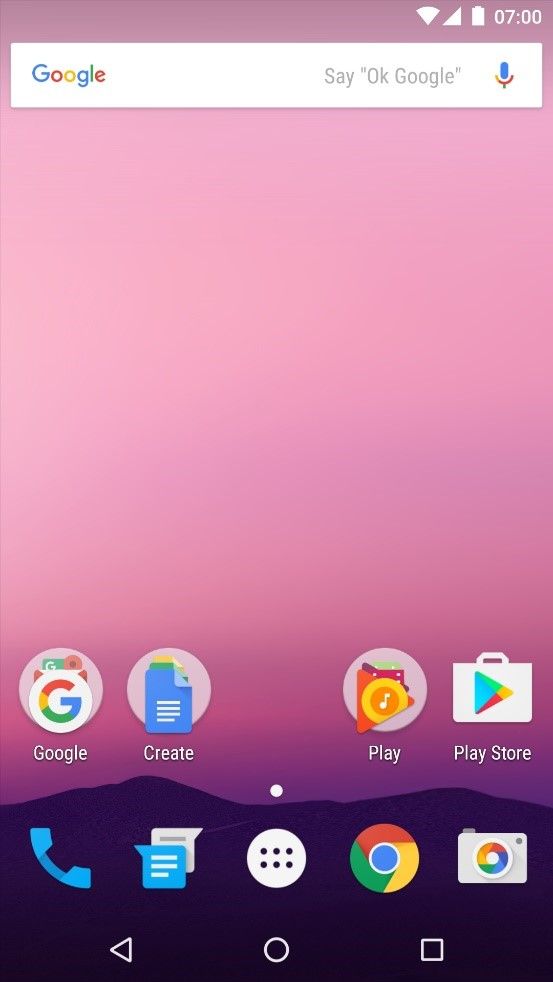This image showcases the screen of a digital device with multiple recognizable elements. In the top left corner, there are three icons: a cellular signal icon, a Wi-Fi icon, and a battery icon indicating the device’s status. Adjacent to these icons is the time displayed as 07:00. 

Directly below this, a search bar is prominently featured. Inside the search bar, the text "Google" is positioned on the left, and on the right, it prompts with the phrase "Say 'OK Google'" alongside a microphone icon, indicating voice search capabilities.

The background beneath the search bar is a gradient transitioning from pink at the top to black at the bottom. Below the gradient background, there is a grid of app icons arranged in two columns and two rows. 

The top row of apps, from left to right, includes:
1. Google – likely the main app interface for Google services.
2. Create – possibly a productivity or art-related app.
3. Play – an entertainment or media app.
4. Play Store – the app for accessing and downloading other applications.

Directly beneath, the bottom row of apps include, from left to right:
1. A blue phone icon, representing the phone app used for making calls.
2. An app represented by a quotation marks icon, likely indicating a messaging or comments app.

Overall, the screen provides a quick overview of common functionality with clear visual organization.